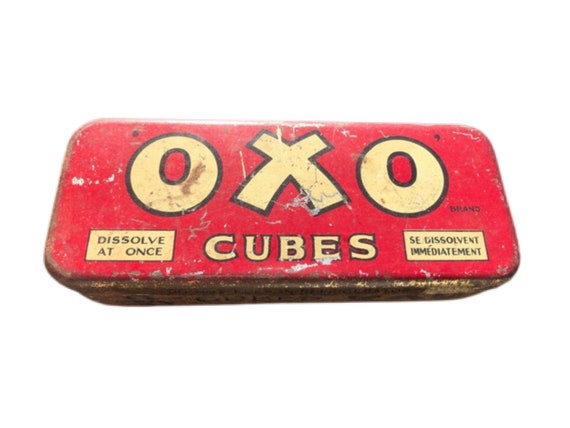The image features an old, worn red metal tin, displayed against a solid white background. The tin is rectangular with curved corners and shows significant rust and wear, with chipped paint and numerous scratches. Prominently displayed on the tin in large, block yellow letters outlined in black is the word "OXO." Beneath this, in black text within a rectangular yellow spot, it reads "dissolve at once." Adjacent to it is another text in black saying "C-dissolvent immediatement," indicating the product’s dissolving properties in both English and French. The tin, once bright red, now has areas where the paint is missing, revealing the metal underneath. Despite its age and condition, the tin’s historical branding and messaging remain partly legible.